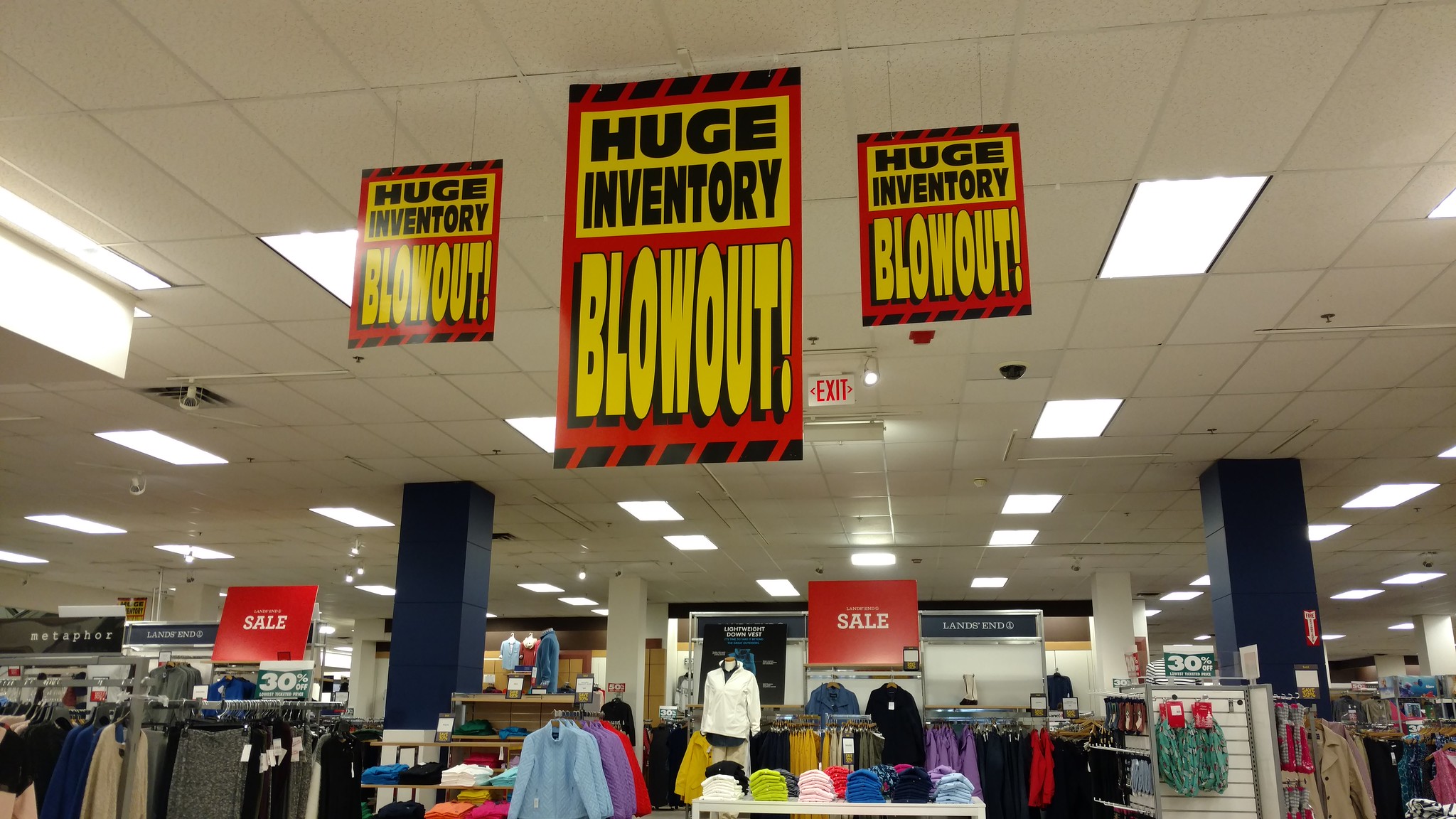This photograph captures the interior of a retail store, showcasing a detailed view from ceiling to floor. The ceiling consists of white, rectangular tiles interspersed with rectangular fluorescent lights, providing ample illumination. A small square exit sign with a white background and bold red "EXIT" text is visible. 

Below, the shelves are neatly stocked with an assortment of clothing, including folded shirts, long-sleeved shirts, and skirts, catering to both male and female customers. Vibrant sales signs are prominently displayed, hanging from the ceiling. These red and yellow square signs announce a "HUGE INVENTORY BLOWOUT," with the word "BLOWOUT" highlighted in yellow, accompanied by an exclamation point in a bold, impactful font. Additional signs indicate a 30% discount, enticing shoppers with attractive deals.